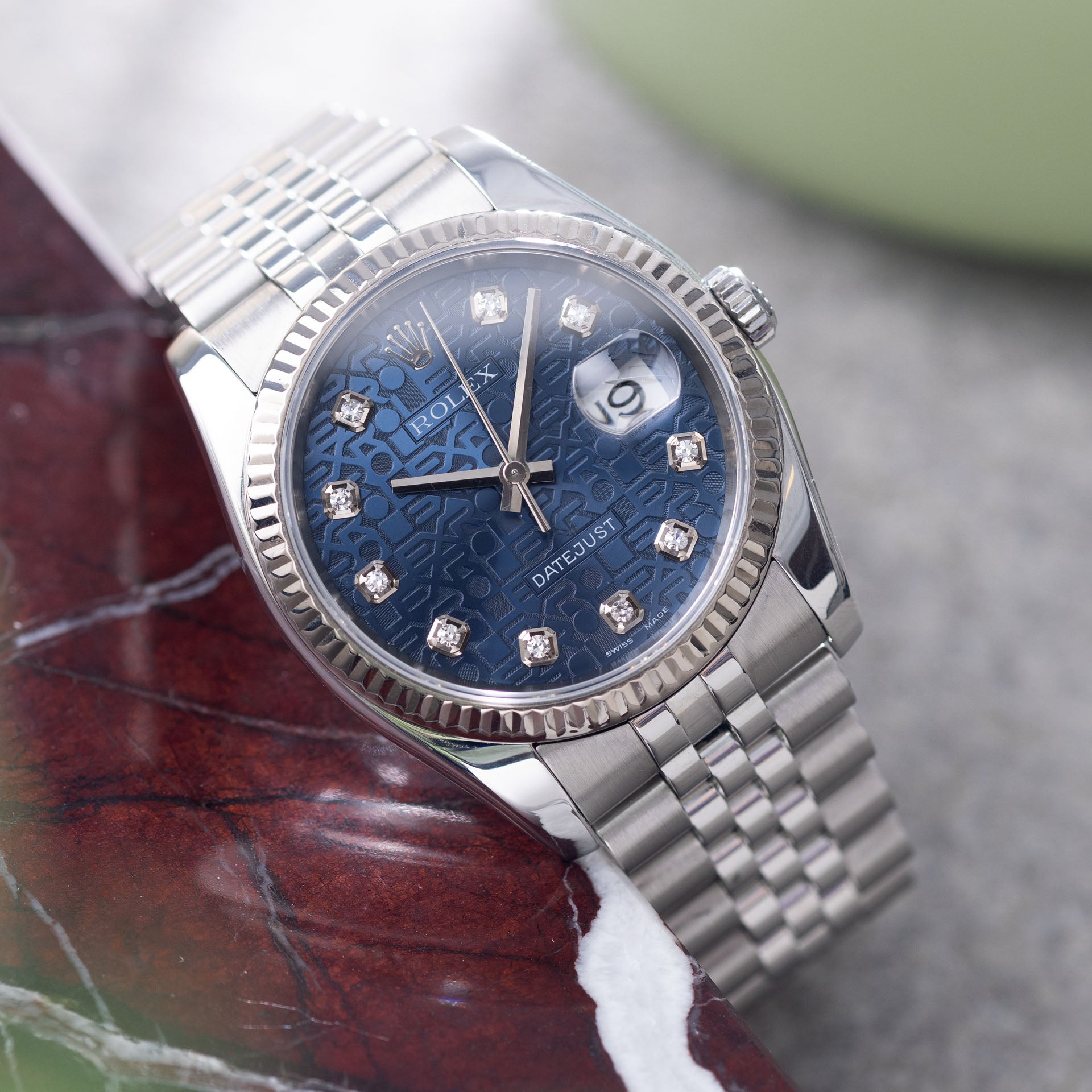The image showcases a detailed close-up of a silver Rolex watch featuring a striking blue face. The watch is positioned diagonally from the upper left to the bottom right of the image. The hour, minute, and second hands are a sleek silver-gray, and the hour markers are replaced with diamonds set in square prongs. Below the 12 o'clock mark, "Rolex" is inscribed, while above the 6 o'clock mark, it reads "Datejust." 

A date window at the 3 o'clock position displays the number 19. The watch's band is wide and silver, complementing its overall elegant design. The winding and adjustment knob is located on the upper right side of the watch face. The background consists of a mix of colors and textures: red and black material on the left side, a gray area immediately below the watch, and an out-of-focus green area at the top right, creating a contrasting backdrop to the luxurious timepiece.